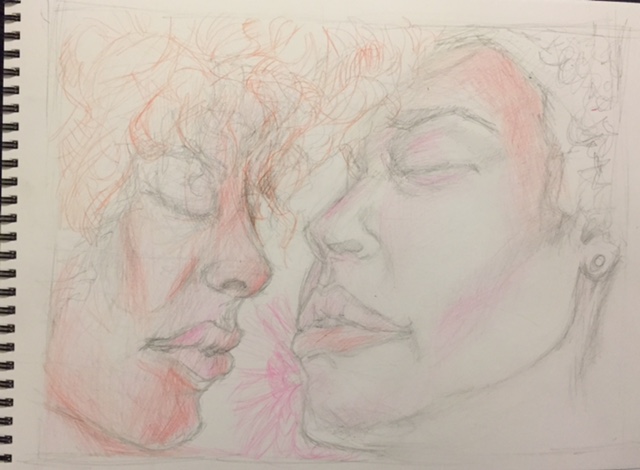This detailed photograph features a sketchbook drawing on plain white paper, showcasing a complex and intriguing scene. On one side, a face is meticulously drawn using shades of peach and pale pink. The person’s pale pink lips, delicate nose, closed eyes adorned with eyelashes, and wisp of gray and orange hair suggest a refined yet subtle aesthetic. Their chin is delicately outlined, contributing to the overall gentle appearance.

Adjacent to this face, another person’s visage appears, with the two faces almost touching, creating an intimate atmosphere. Pink lines artistically connect the characters' mouths, enhancing the closeness between them. The second face also displays closed eyes, highlighted by pale pink shadowing and delicate gray eyebrows. Subtle pale red and pink tones contour their face, emphasizing their full, pinkish lips and visible nostrils. An earring dangles from their ear, adding a touch of elegance to the character. Wisps of hair lightly frame their face, and a slight double chin is discernible.

The background is filled with scattered black spirals and scribbles, adding a layer of complexity and dynamism to the drawing. The artist employs pencil for the primary sketching, capturing intricate details that provide depth and a lifelike quality to the depicted scene.